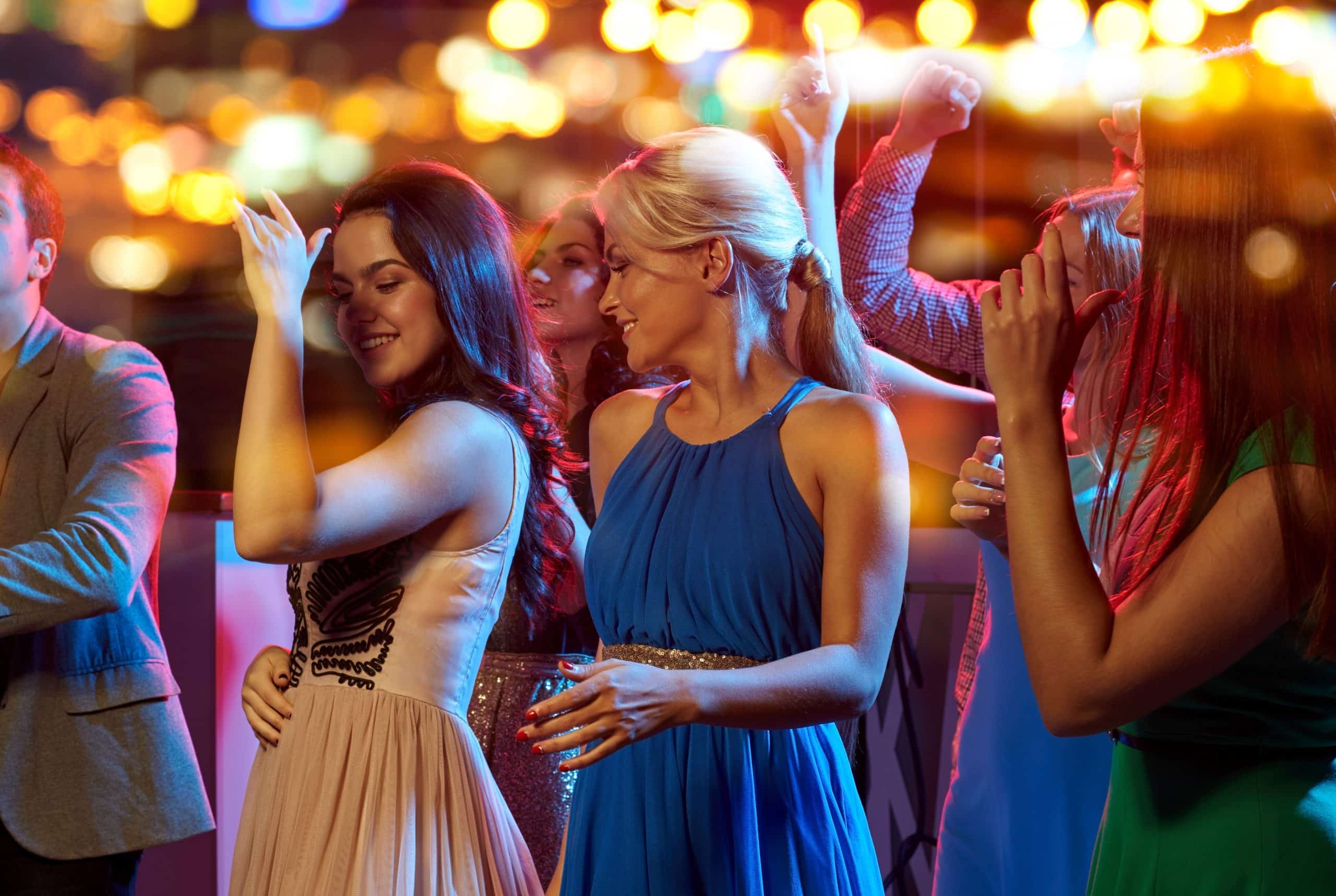This detailed photograph captures a dynamic and lively scene at what appears to be an indoor music festival, featuring vibrant dancing and a warm ambiance. The primary focus is on two young women of Caucasian descent, centered in the frame amidst a backdrop of softly glowing white and amber-colored lights hanging overhead. 

On the left is a brunette with long, slightly wavy hair that exhibits a hint of purple due to the surrounding lights. She is wearing a sleeveless, blush-toned cocktail dress adorned with brown beads at the bust, which flares out at the waist. She strikes a captivating pose with her right hand resting on her stomach and her left arm bent at the elbow, palm facing outward. 

Next to her stands a blonde woman with her hair pulled back in a ponytail, donning a halter-style blue pleated dress with a silver waistband. She is intently watching her friend and mimicking her dance moves. Alongside and behind them, more dancers can be seen, including a glimpse of a man in a light brown dress jacket on the far left. The overall atmosphere of the photo is lively and festive, filled with the energy of people dancing under the enchanting display of hanging lights.